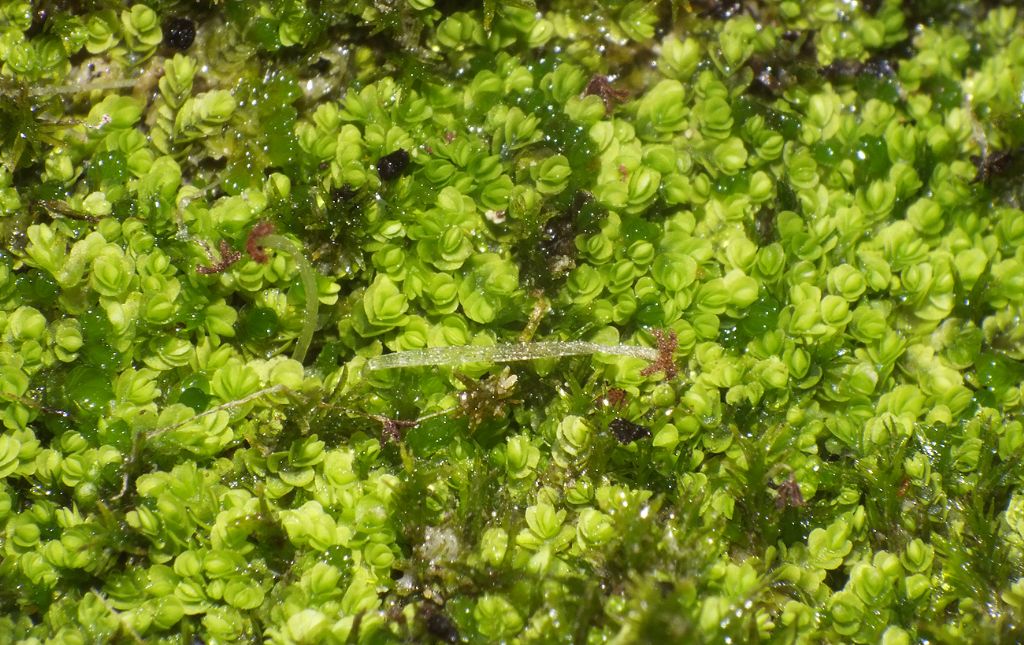The image showcases a vibrant cluster of small, lemon green leaves in varying shades of light and dark green. These leaves exhibit a round, rosette-like formation reminiscent of miniature cabbages, each glistening with numerous water droplets. Scattered among the leaves are dark brown flowers, their numbers significantly fewer compared to the lush foliage. Adding to the intricate tapestry are delicate sprigs of grass-like plants and a few translucent, mushroom-like stalks, creating an impression of a thriving miniature ecosystem. The entire scene has a shimmering, wet appearance, suggesting it may have just rained or be situated in a water-rich environment, possibly even underwater. Glistening elements—including a white, silver, and glittery line with a red tip—add a touch of mystery, hinting at the presence of a sea creature or marine organism. The tableau is a detailed interplay of plant life and moisture, evoking the rich, wet vibrancy of a coastal or aquatic setting.